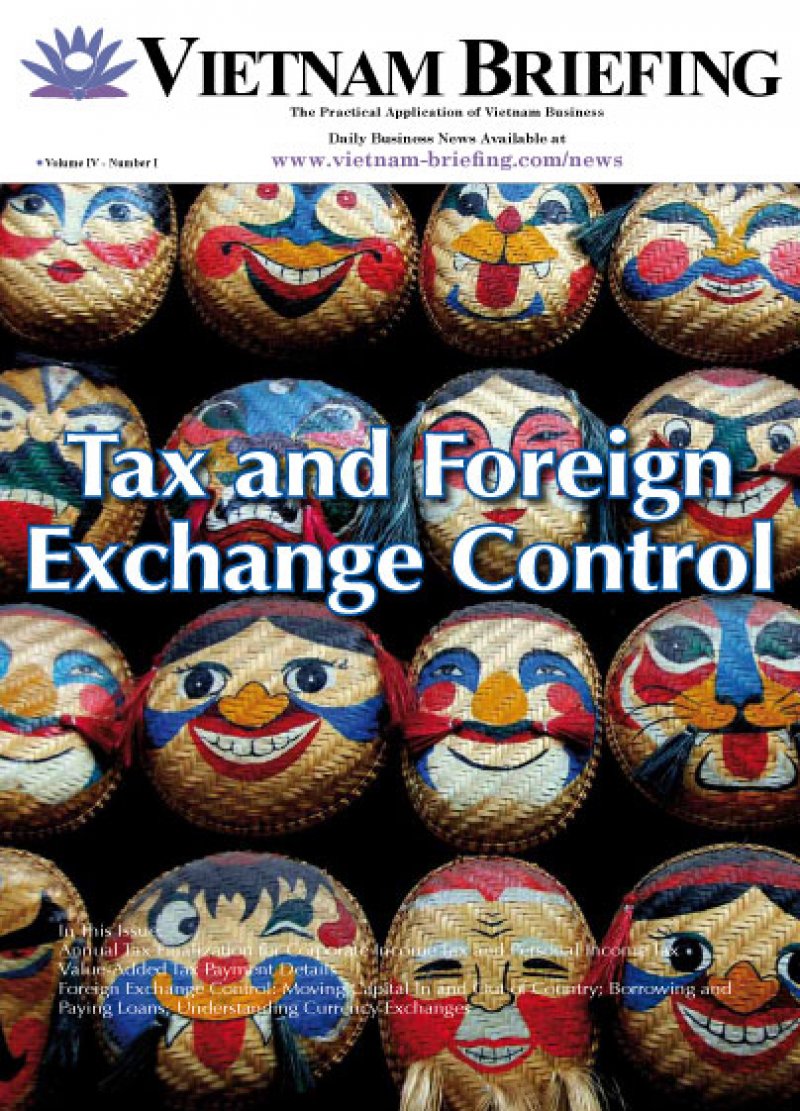This image is the cover of "Vietnam Briefing," a magazine focused on the practical application of business in Vietnam, specifically featuring daily business news accessible at www.vietnam-briefing.com/news. This is Volume 4, Number 1 of the publication. The cover prominently displays the headline "Tax and Foreign Exchange Control" in white text with a blue outline centered on the image. Below the headline, there is a section labeled "In This Issue," which lists various topics relating to business practices such as paying loans, understanding currency exchange, foreign exchange control, moving capital, and borrowing.

The cover image itself is vibrant and eye-catching, featuring numerous colorful and expressive basket masks traditionally used during Vietnam's national holiday, Tet. These masks, painted in vivid hues of red, white, blue, and yellow, show a variety of happy and playful expressions. Some have blue or red eyes, yellow noses, and smiles depicting teeth, while others have simple, broad grins, lending a childlike, almost clownish charm to the cover. The title of the magazine is displayed in bold black text, emphasizing the professional yet lively nature of the publication.